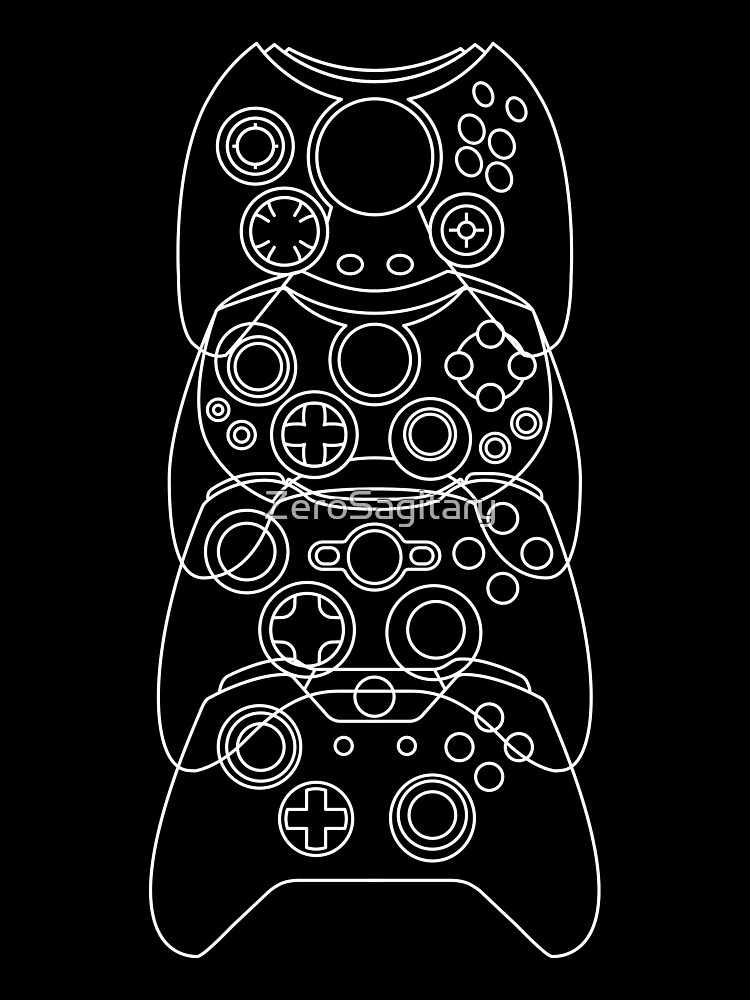The image features a minimalistic, black background with a central watermark that reads "Zero Sagittary." Prominently displayed are four hand-drawn, white outlined video game controllers stacked on top of each other. These simple, see-through outlines reveal the black background beneath them. Each controller, while similar, showcases different directional pads and button layouts reminiscent of classic PlayStation, Sega, and Nintendo designs from years ago. The artistic design emphasizes the nostalgic appeal of these controllers with detailed yet straightforward sketches of knobs, buttons, and directional arrows, capturing the essence of retro gaming.